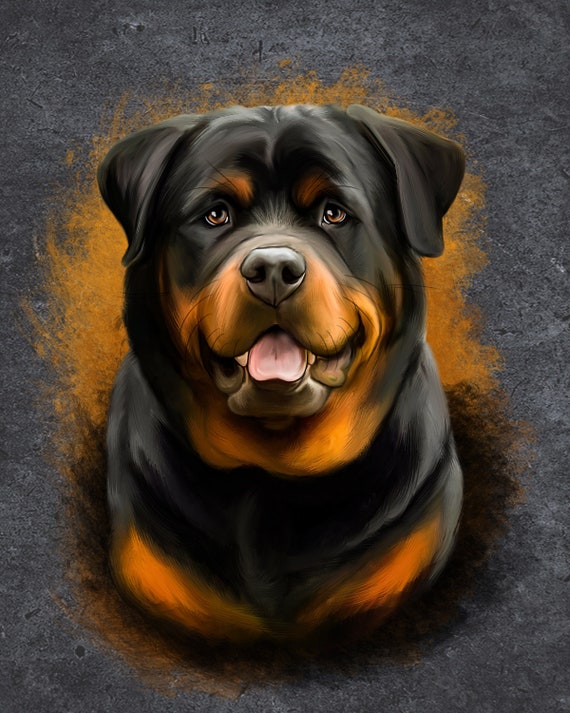The image showcases a highly realistic painting of a happy Rottweiler, captivating with its detailed features. The Rottweiler's face stands out with expressive brown and black eyes glancing upwards, complemented by short, triangle-shaped ears that lie flat. Its tongue and canines are visible as it happily gazes, emanating a joyful aura. The dog’s black fur contrasts beautifully with vivid orange accents on its snout, eyebrows, and chest. Only the portion of the dog from the breast upwards is depicted, with the background transitioning from orange near the head to black below, set against a grey backdrop further enhancing the depth of the painting. This portrayal emphasizes the Rottweiler’s distinct markings and warm presence, making the artwork both adorable and striking.